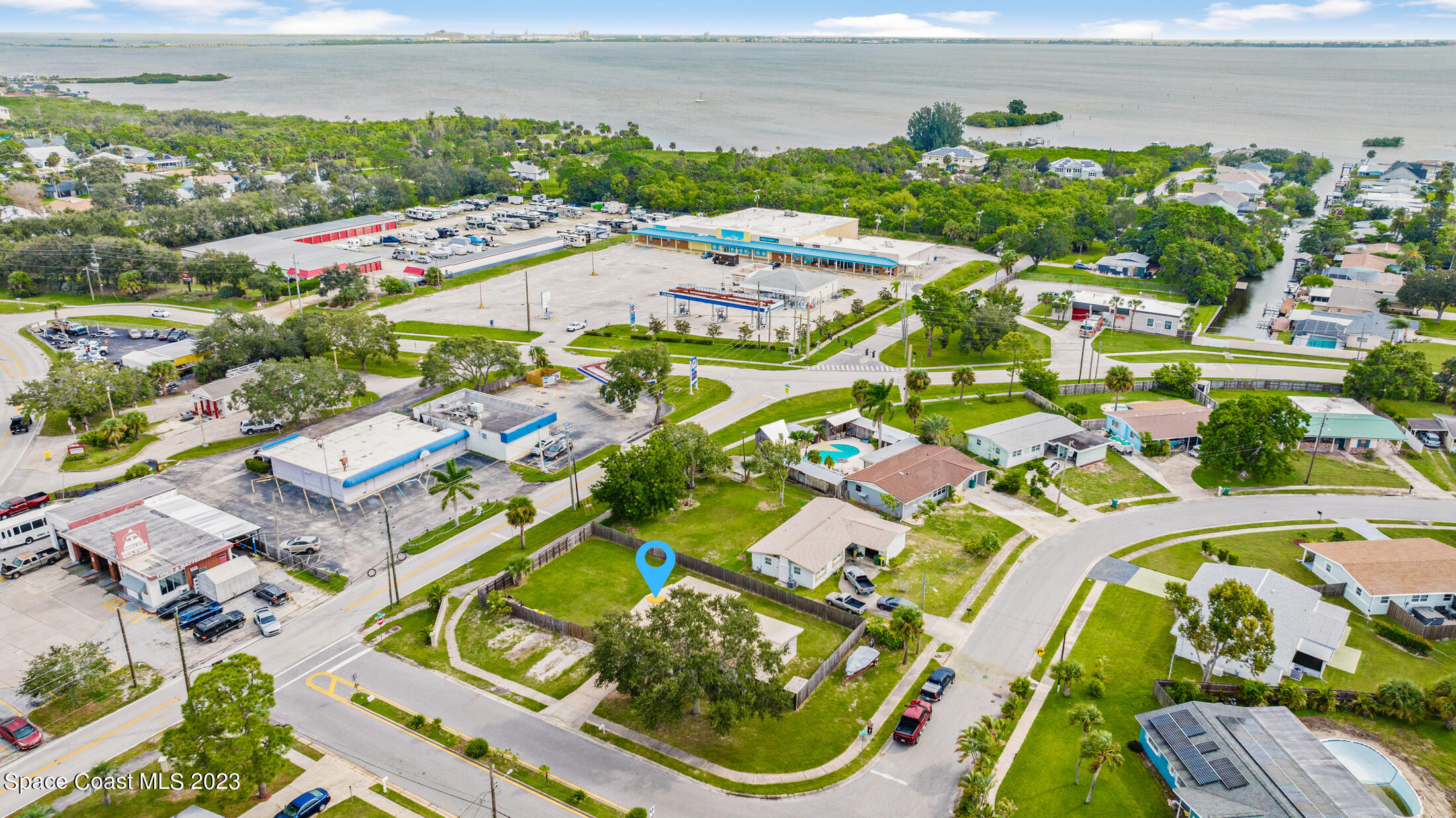This image is an aerial view of a coastal town, displaying a broad landscape that stretches from the bustling town center to the expansive ocean at the horizon. In the top portion of the image, the ocean extends into the distance, hinting at a small island or peninsula on the left. The sky is a clear blue with fluffy clouds scattered throughout. The town itself is vibrant, with a mix of residential, commercial, and natural features. Prominently, there's a large storage facility identifiable by its orange doors, and adjacent to it, a notable building with an expansive porch area flanked by electric car chargers, possibly indicating a gas station or service area.

Across the street, a Marathon and a Chevron station stand out, surrounded by several houses. Along curved streets, some homes feature swimming pools—although one is notably empty. The residential area continues towards the coastline, dotted with various deciduous and palm trees, creating a lush backdrop. There are also roadways interweaving through the town, leading to parking lots and driveways filled with automobiles. 

A blue locator symbol is positioned in the bottom middle section, highlighting an area of green trees, and the caption "Space Coast MLS 2023" is visible in the bottom left corner, indicating the image's timeframe and relevance. The detailed depiction includes two individuals walking on a rooftop and various smaller identifiable infrastructure elements, all contributing to a comprehensive overview of this picturesque coastal town.